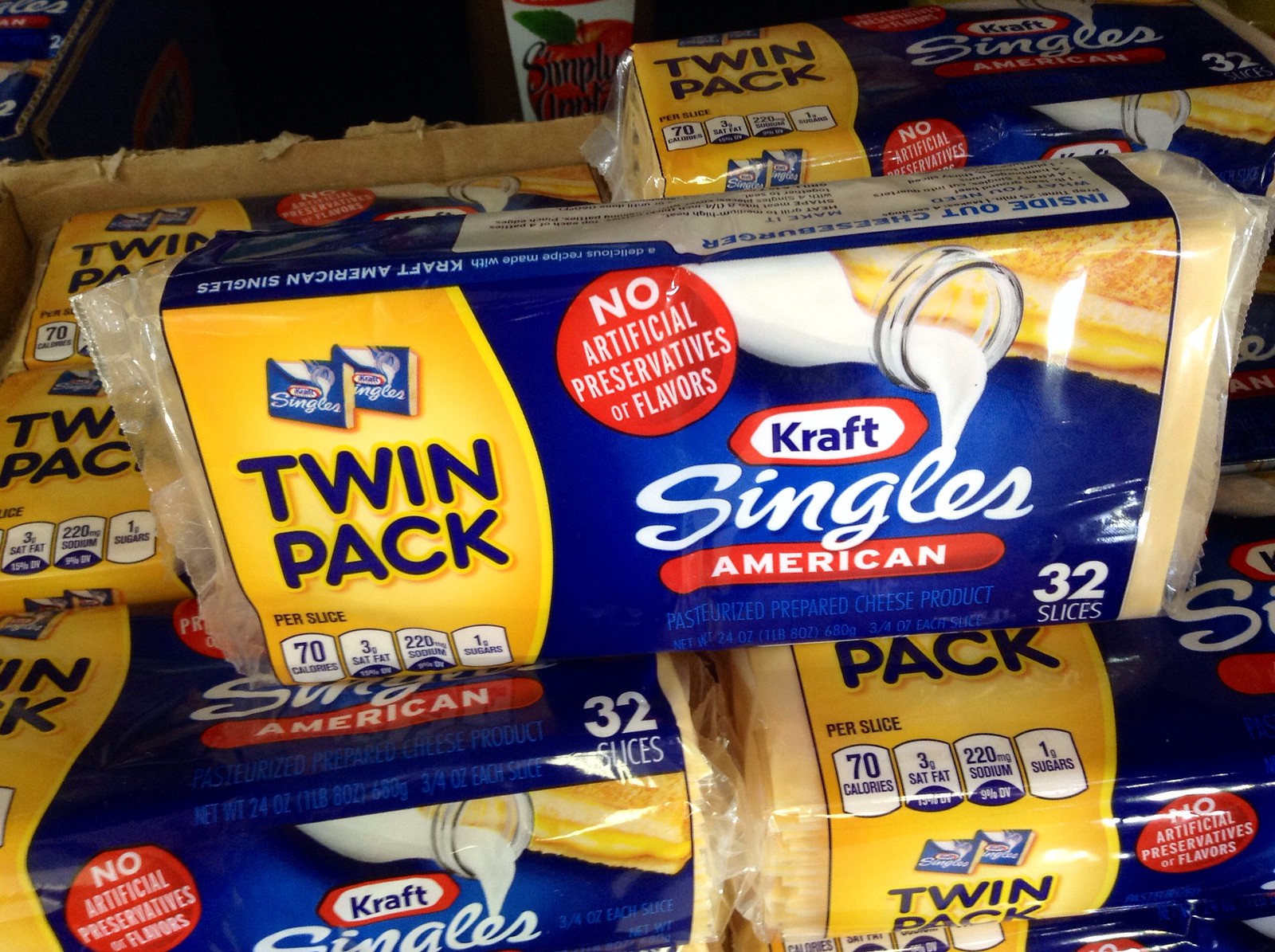This square image showcases multiple packaged products, all bearing a similar appearance. At the center of the composition is a prominently featured rectangular package. The labeling on the front of this central package provides detailed information: on the left side, it states "Twin Pack," and beneath that, "Per Slice." Further down, it indicates "70 calories." Moving to the right side, the label reads "3g Saturated Fat," followed by some smaller, illegible text due to blurriness. Additionally, at the rightmost side of the package, it specifies "No Artificial Preservatives or Flavors." The product in focus is "Kraft Singles American." This central item stands out amidst the surrounding similar products.